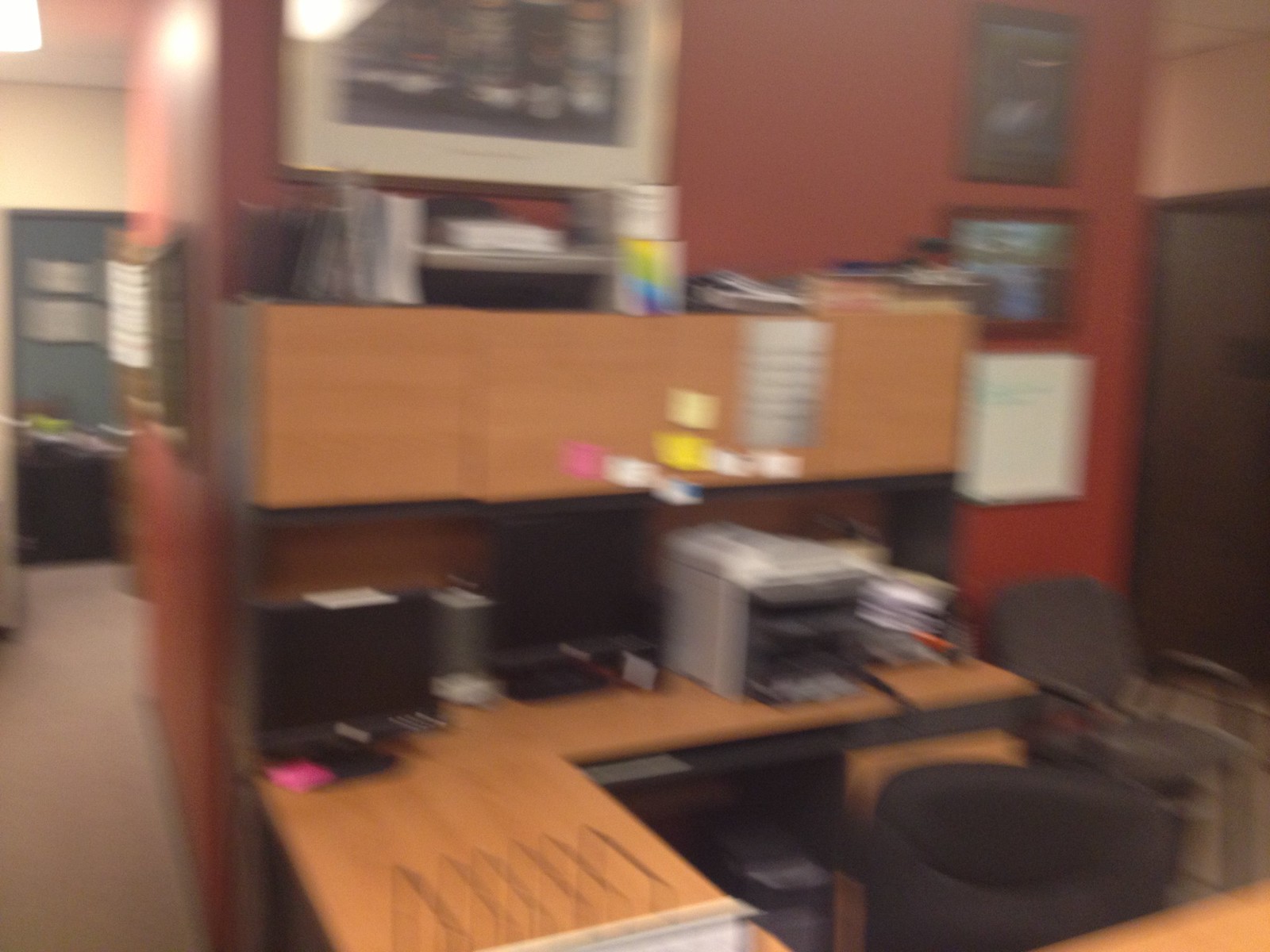The image depicts a somewhat generic and cluttered office space with various elements contributing to the overall disarray. Dominating the foreground, there is a U-shaped desk with a brown wooden surface and a black framing, which features an upper shelving area in matching colors. Although the image is of poor quality and somewhat blurry, it is possible to make out several details. The desk accommodates a few computer monitors, a speaker between them, a printer, and a stack of papers. Towards the left side, the desktop is extended in an L-shape. 

Higher up, there is a CRT monitor perched on a shelf too high for regular use, alongside other stored items such as papers and envelopes. Among the decorations on the wall, notably to the right, there are several framed pictures as well as possible calendars or chalkboards. The workspace also includes an office chair, some vertical wire trays for papers, and what appears to be trays or dividers that may be intended for printer use. The shelving unit onto the wall features cabinet doors and various colored post-it notes (pink, white, yellow, and darker yellow) adhered to it. The entire scene suggests a busy, albeit slightly messy office setup, possibly within a home office given some of the mixed-use furnishing elements.